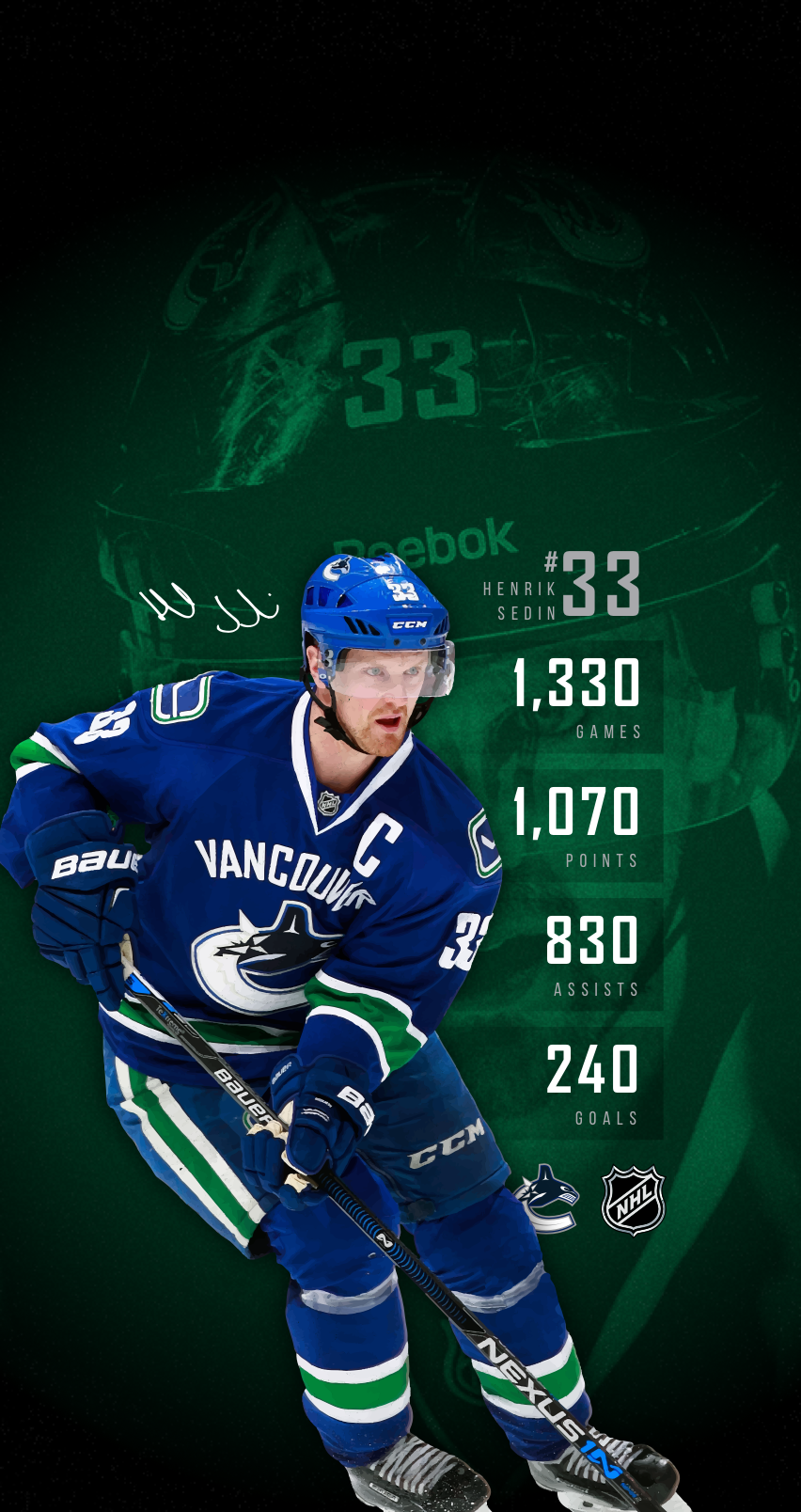The promotional image features NHL ice hockey player Henrik Sedin against a green background. The foreground displays Sedin in full hockey gear, with his blue uniform bearing the "Vancouver" logo and additional logos and text. His uniform includes patches from CCM and his stick is emblazoned with "Nexus." Sedin is depicted in action, skating and holding a black hockey stick. To his right, key statistics are listed in white font, including "Henrik Sedin, number 33, 1,330 games, 1,070 points, 830 assists, 240 goals." The background also includes a close-up image of Sedin’s face, overlaid with a green filter, and his signature appears above his head. A black badge with a white outline displaying the NHL logo is positioned below the stats.